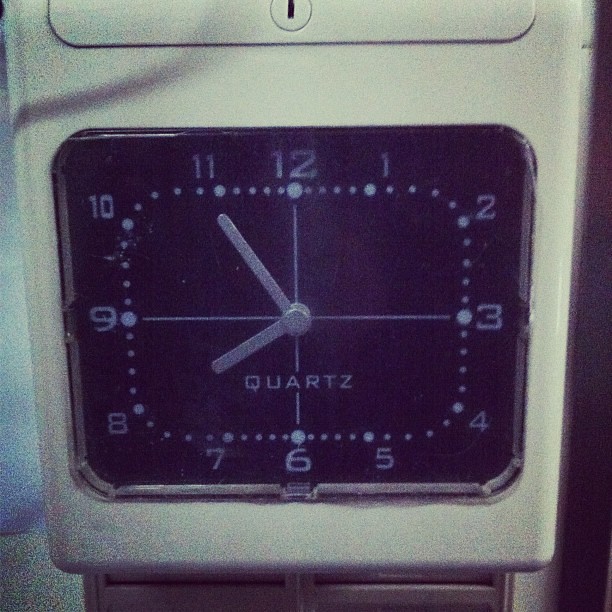The image depicts a vintage, low-resolution photograph focused on an antique timepiece, possibly a clock or watch, characterized by its close-up view. The timepiece features a unique square, cream-colored face with a contrasting black inner dial. Surrounding the dial are numeric markings from 1 to 12, arranged in an unconventional, grid-like pattern due to the square shape of the face. The numbers 2, 3, and 4 are aligned vertically on the right, while 10, 9, and 8 are vertically aligned on the left. Similarly, the numbers 7, 6, and 5 are horizontally placed at the bottom. Beneath the dial, there appears to be a brown band, suggesting the timepiece might be a watch. The photograph has a nostalgic, vintage quality, lending a sense of timeless charm to the intricately detailed timepiece.